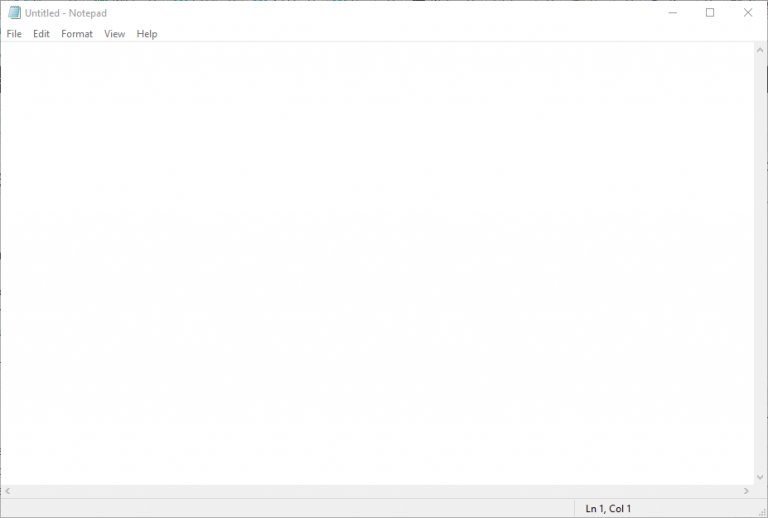The image captures an almost barren web page interface. In the upper left corner, there is a small icon of a blue notebook. To the right of this icon, "Untitled - Notepad" is displayed in text. Beneath this, a horizontal menu bar includes the following options: "File," "Edit," "Format," "View," and "Help," each spaced about an inch and a half apart. In the upper right corner, the window control icons are lined up: a minimize button, a maximize/restore button, and a close button (X). The main portion of the page is entirely blank and white, spanning about eight inches downward. The only other text present is located in the lower right corner, displaying "Ln 1, Col 1."